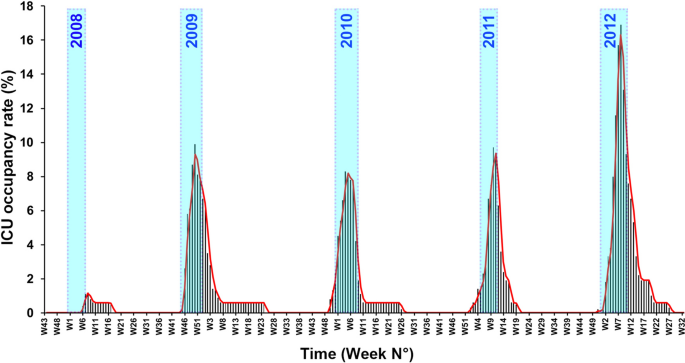The image is a detailed bar graph illustrating ICU occupancy rates as a percentage, ranging from 0 to 18% on the vertical axis. The horizontal axis displays weekly intervals from the years 2008 to 2012. The graph confirms that ICU occupancy was consistently measured each year, highlighting a particularly notable increase in 2012, which exhibits the highest rate of all the years depicted. The trend suggests a rise in ICU admissions over the time period, emphasizing the strain on healthcare systems and the increasing severity of patient conditions over these five years.